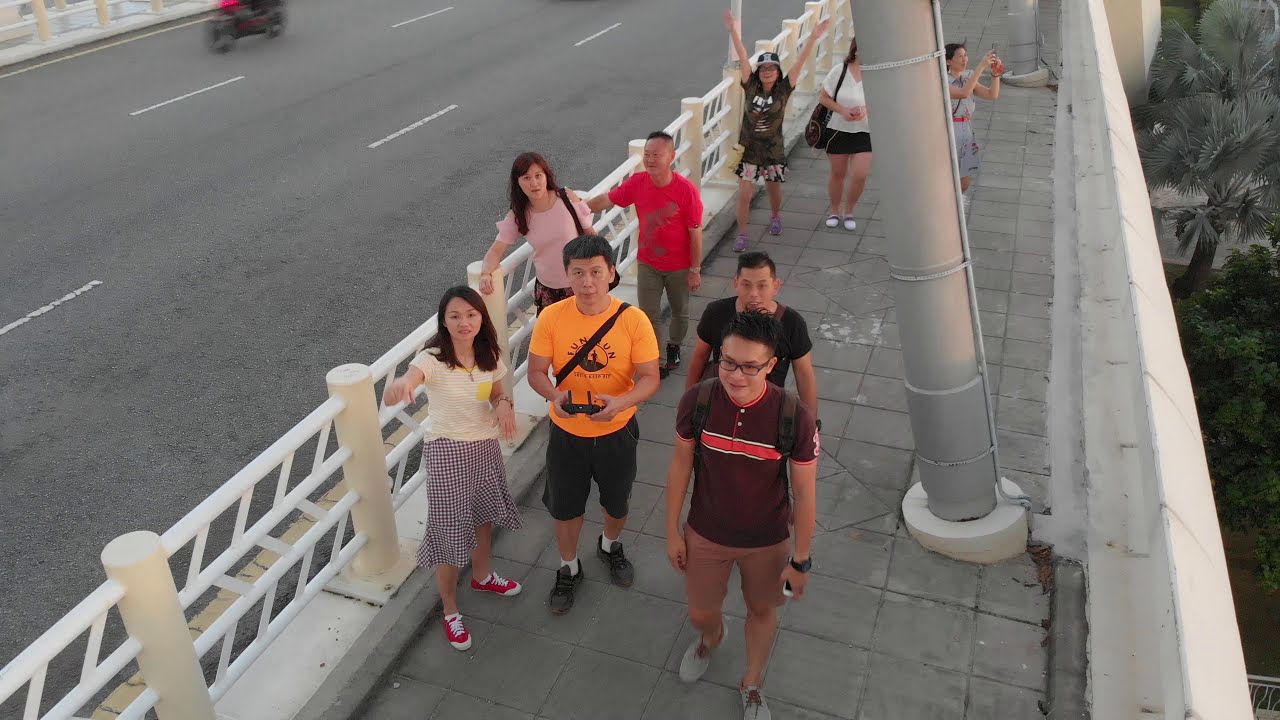The photograph, taken outdoors during the day, depicts a group of people walking on a stone-tiled walkway alongside a three-lane bridge. The right side of the bridge features white barriers separating the walkway from the road. In the top left corner of the image, a motorcycle can be seen peering into the frame. At the center front of the group, a young woman in a checkered skirt, red shoes, and white shirt points at the camera. Beside her, a man in a yellow t-shirt with a black strap across his shoulder, black shorts, and black sneakers operates a remote control, likely for a drone taking the picture. Next to him stands a young man in glasses, wearing a brown shirt with a red or orange stripe and brown shorts, accompanied by another man in a black t-shirt behind him. Against the railing separating the walkway from the street, a woman in a pink shirt with long hair leans, with a man in a red t-shirt standing behind her. Further back, three women are seen: one in a dark shirt, shorts, and a baseball cap has her arms raised in triumph, another in a white shirt and black shorts stands beside her, and a third woman in a bluish dress is taking a photo over the edge of the bridge. The image, rich in natural light, captures the vibrant colors and the lively scene clearly.